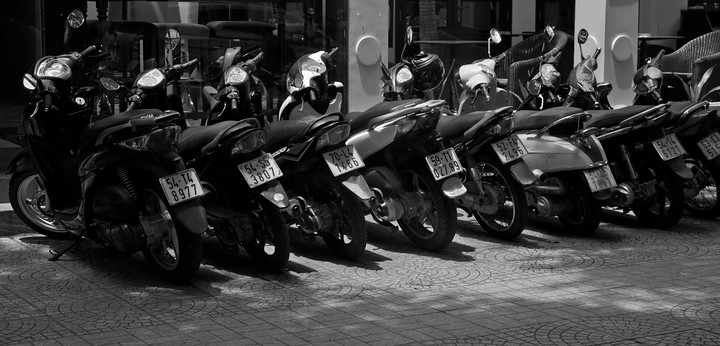A black and white photograph in a rectangular landscape orientation depicts a line of parked motorcycles facing away from the viewer. The motorcycles are aligned on a brick street that features intricate patterns, capturing a distinctive noir aesthetic. Each motorcycle is adorned with a white license plate, several of which are visible and legible. The first license plate reads "54-T48977," followed by "54-553807," "70L41456," "59T102789," "54F42496," "54S5 3807," and a partially legible "631351." The motorcycles are predominantly dark in color, with some having silver accents, such as the side bumpers and handlebars. They are parked in front of a building adorned with two large white columns and windows running across its facade. The photograph captures the scene from behind the motorcycles, highlighting their symmetry and uniformity, with each set of handlebars slightly tilted to the right. The sun appears to be shining, casting a gentle light that adds to the nostalgic and classic feel of the image.